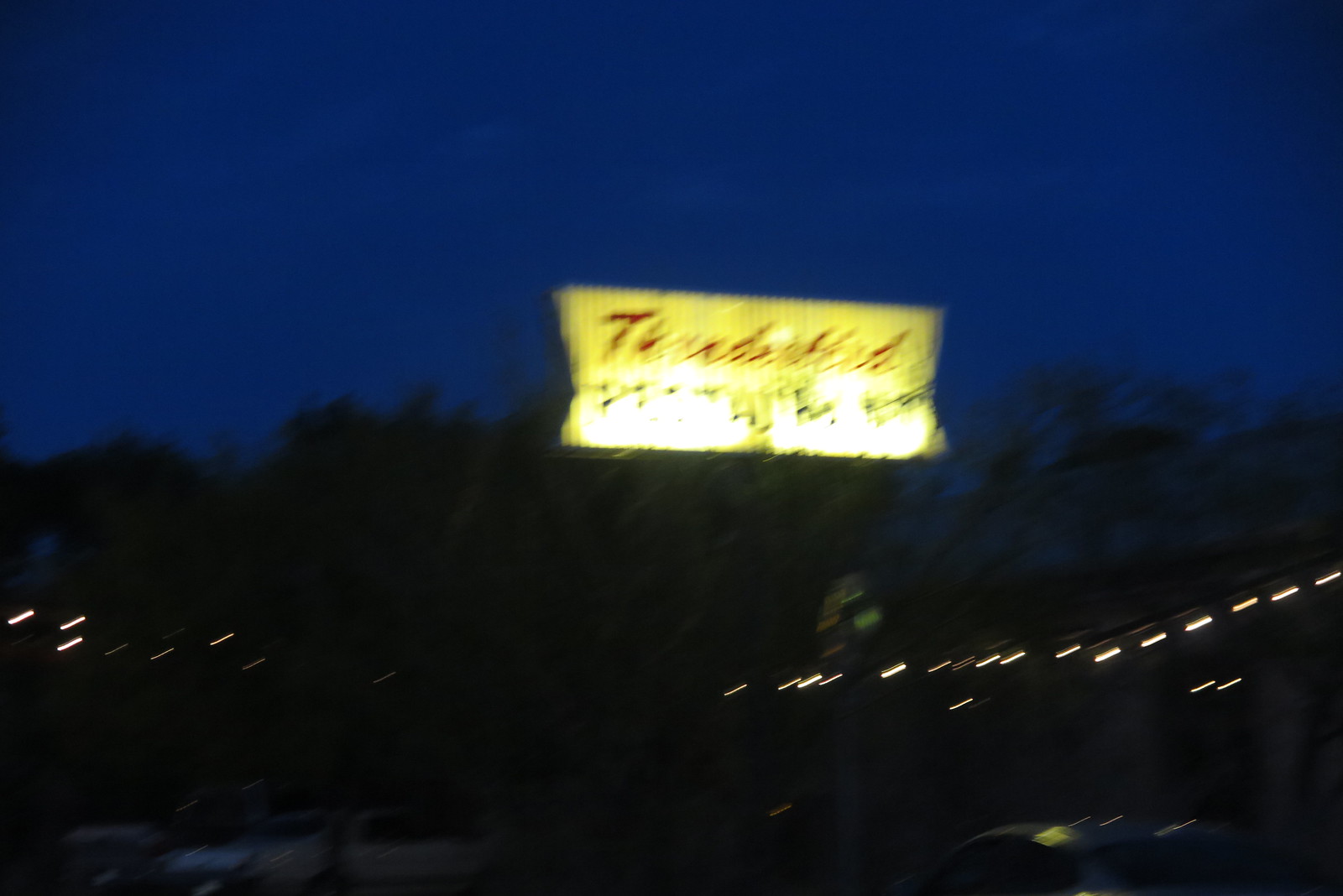A blurry nighttime photograph captures a classic, old-fashioned marquee or billboard. The illuminated sign, possibly reading "Thunderbird" or something similar in cursive lettering, exudes a vintage charm. The image is unfocused due to the motion of a moving car. Small lights dot the roadside, adding to the ambiance. The sign itself is lit by external ground lights, which cast an upward glow that only highlights the bottom portion, leaving the top in shadow. This creates a glare that partially obscures additional text on the sign, rendering it unreadable.